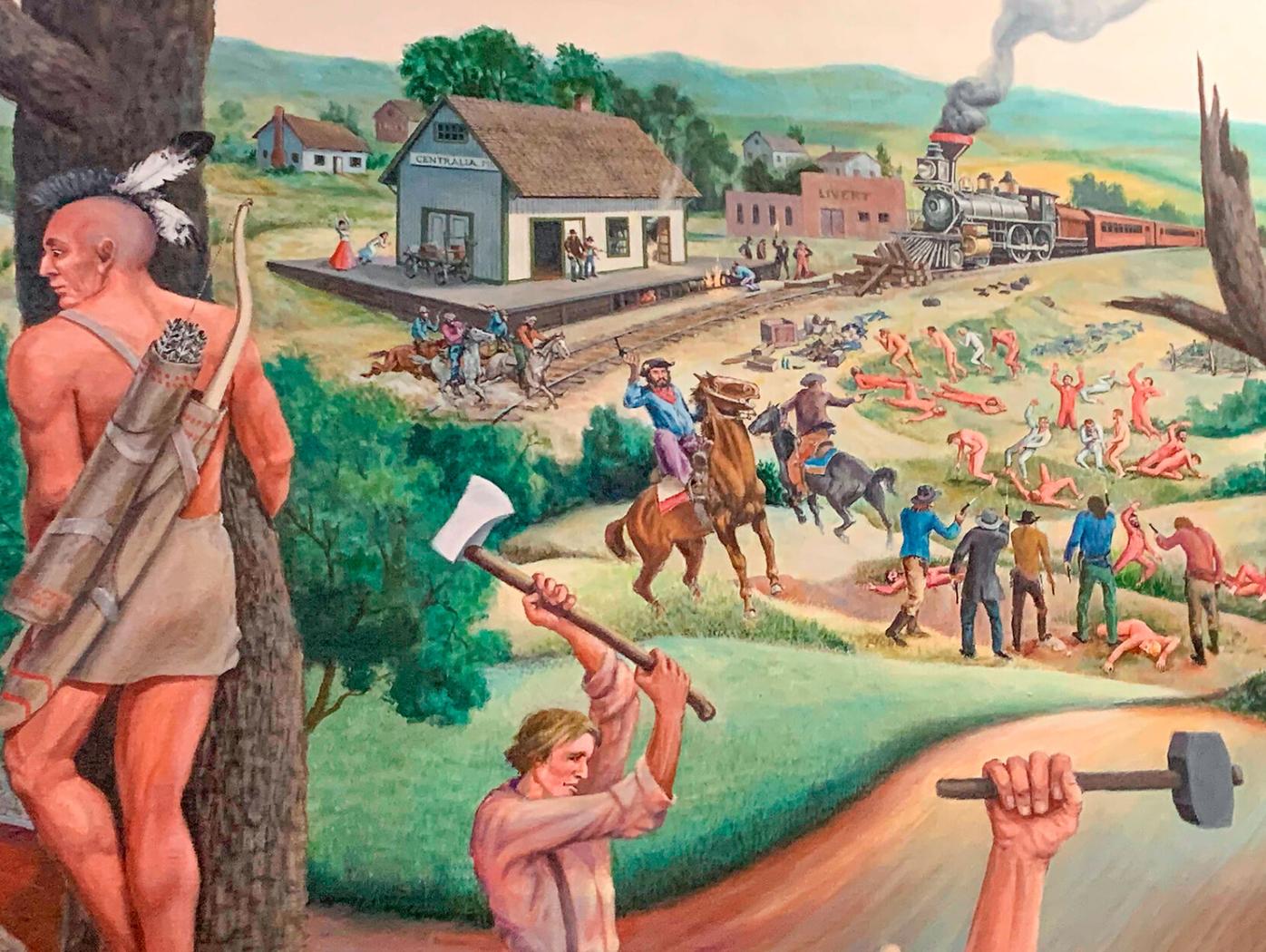This detailed color illustration, likely created using colored pencils, depicts a chaotic outdoor scene filled with intense action and emotion. On the far left, partially hidden behind a tree, is a Native American man with a mohawk and two black and white feathers adorning the back of his head. He is armed with a bow and has a quiver of arrows strapped to his back, dressed only in a beige loincloth, and has an expression of despair while looking off to the left. 

In the foreground, a man raises a hatchet high in the air, ready to strike, while to the lower right, there is a disembodied hand clutching a sledgehammer. The background reveals a train labeled "Centralia" pulling into a station, belching dark gray steam. The train is silver metallic in front with reddish-orange carts. Near the train tracks, a man desperately tries to extinguish a fire. Surrounding the train and the station are numerous figures: men on horseback wielding guns, people in red Union suits—some standing with their hands raised, others lying on the ground, and what seems to be dead bodies scattered about.

Additionally, two men on horseback appear to be shooting at the people in red Union suits, adding to the turmoil. In the background, various structures, including buildings and houses amidst green trees, set the scene, while train tracks cluttered with wood indicate further disruption. This image vividly captures a scene of conflict, tension, and despair, underscored by the varied emotional responses and chaotic activity throughout.